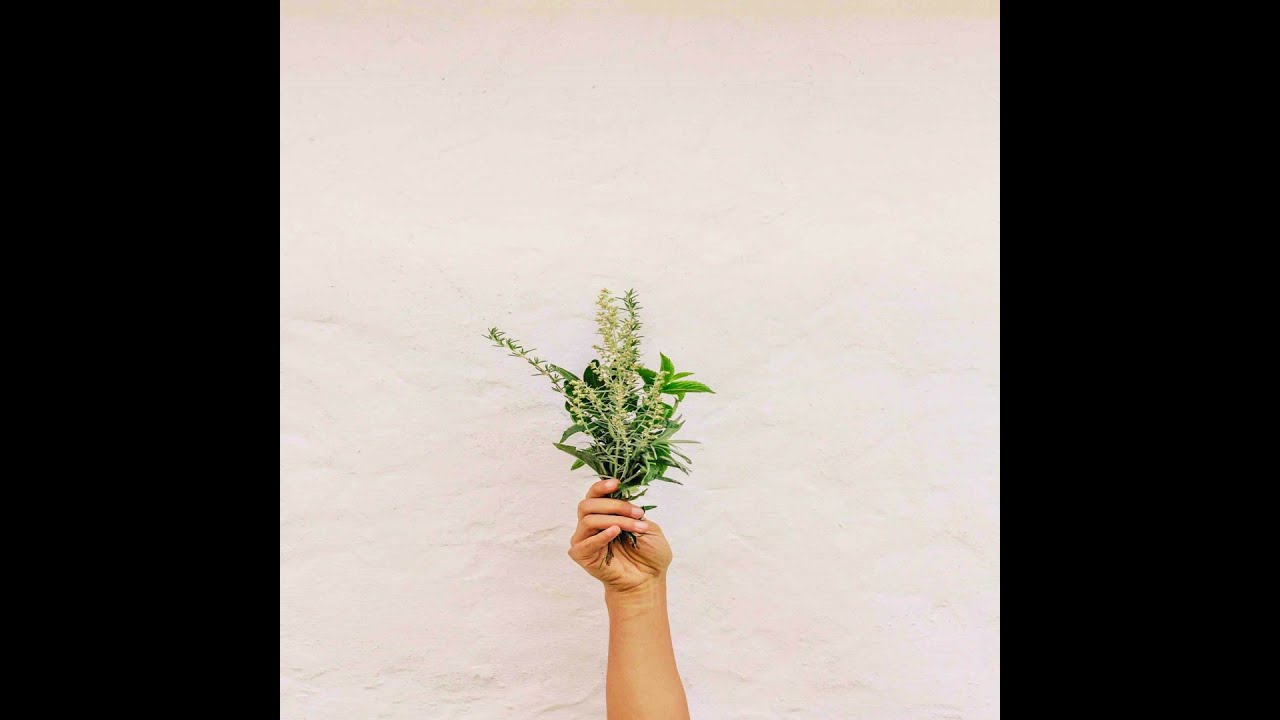In this detailed photograph, a tan hand, which appears to be a woman's, extends upwards from the bottom of the frame, reaching towards the middle. The forearm is visible, leading to a hand firmly grasping a small bouquet composed of green leaves and delicate, tiny flowers on stalk-like stems. Notably, the pinky finger is stretched straight, while the index, middle, and ring fingers curl around the foliage, and the thumb remains out of view. The background is a textured, off-white stucco, suggesting an outdoor wall. The entire image is flanked by thick black borders on the left and right sides, adding to the composition. The skin complexion of the hand is light brown, though the photo appears slightly compressed, giving the hand a somewhat distorted, squished look.